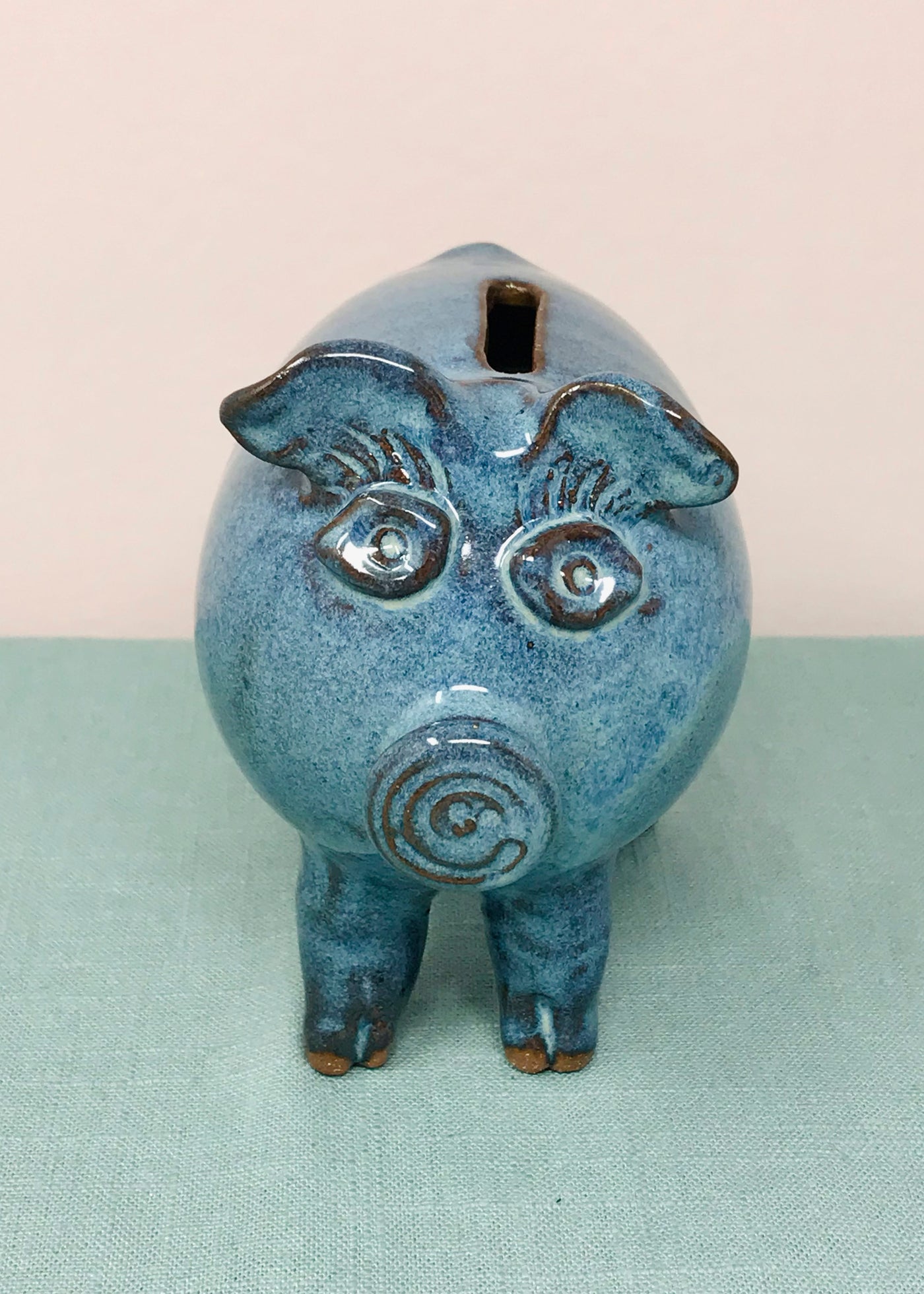The image depicts a ceramic piggy bank shaped like a pig, poised on a light foam green cloth-covered surface with a white or light off-white backdrop. The piggy bank has a distinctive shiny, dark blue or bluish-marble color adorned with brown markings around its eyes, snout, hooves, and trims. Its eyes are designed to appear wide and open, creating an almost soulful expression as it looks directly at the camera. There is a coin slot on its back for inserting coins. The overall image is clear, bright, and well-lit, showcasing the unique details and features of the piggy bank.